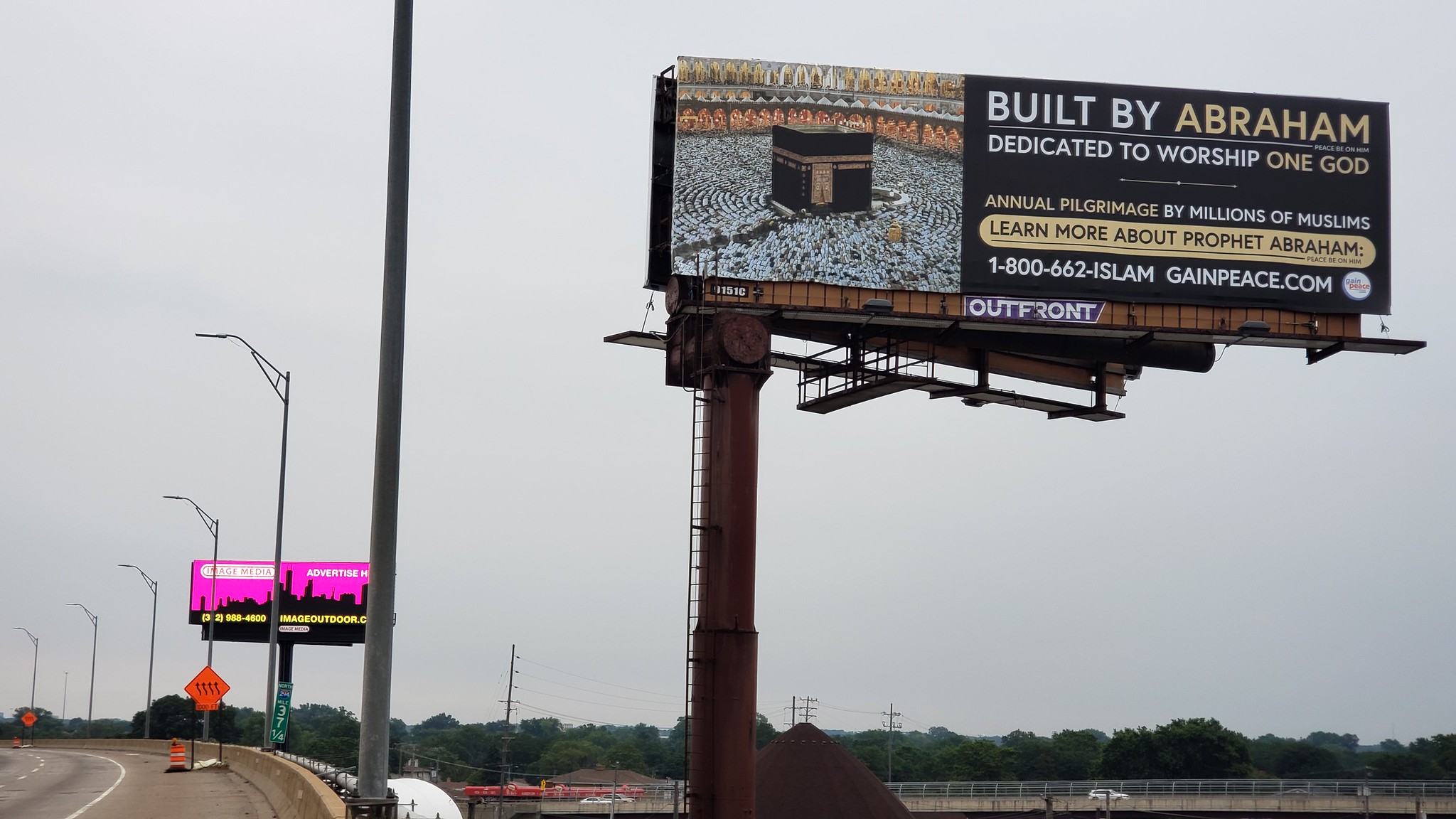This photograph captures a large rectangular billboard prominently displayed along a concrete highway. The left third of the billboard features a central black box set against a backdrop of white, gray, orange, and black hues. The right two-thirds of the billboard boasts a striking black background, adorned with text in tan and white. At the top, the text reads, "Built by Abraham," followed by the phrase, "Dedicated to Worship One God." Beneath this, within a long rectangular tan box with curved edges, black lettering invites viewers to "Learn more about Project Abraham." Anchoring the bottom left of the billboard is a large, wide, brown metal pole, while gray metal supports are visible beneath the structure. Below and behind the billboard, a row of trees adds a touch of natural greenery. To the left, steel poles of streetlights and the edge of a concrete highway are visible, all set against a backdrop of a gray, overcast sky.